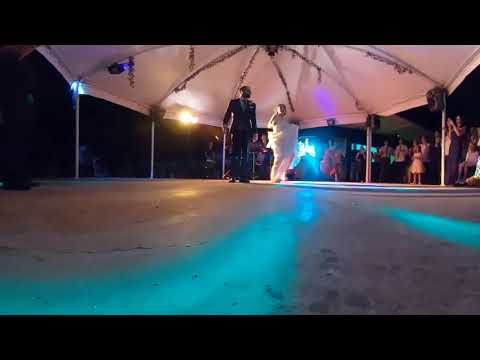In this color photograph taken at night, a bride and groom are captured sharing their first dance on a spacious, gray concrete floor illuminated by a soft blue light. The bride, positioned on the right, is dressed in a flowing white bridal gown, while the groom, on her left, is in a crisp blue suit. Above them, a large white tent ceiling with multiple white support poles stretches out, creating an enchanting canopy. Surrounding the floor, a crowd of wedding guests in formal attire watches the couple with rapt attention. There are bright lights attached to the tent structure, adding a soft glow to the scene. In the distance, a green light from another venue can be seen, adding an additional layer of ambiance to this magical wedding moment.